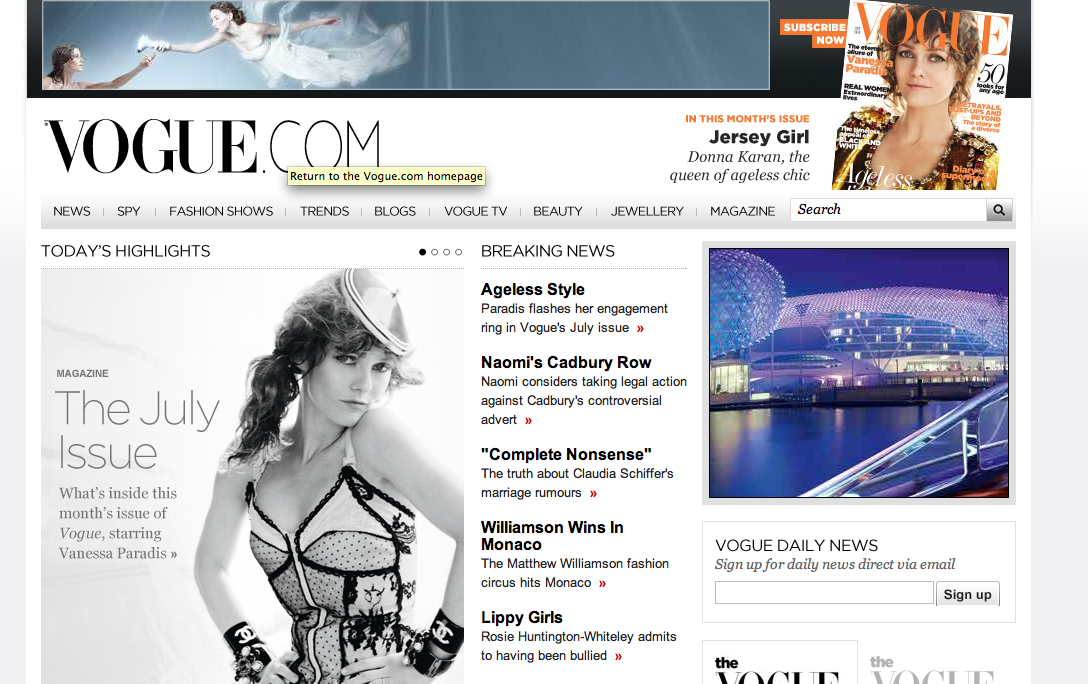**Detailed Caption:**

The image is a screenshot from Vogue.com, prominently featuring the website's header and various navigation options. Near the upper left-hand corner, a small pop-up message appears, displaying the text "Return to the Vogue.com homepage." 

On the upper right-hand corner, the cover of a Vogue magazine is visible, with the headline "In This Month's Issue: Jersey Girl Donna Karan, The Queen of Ageless Chic." Surrounding the website header, there are several clickable buttons labeled: News, Spy, Fashion Shows, Trends, Blogs, Vogue TV, Beauty, Jewelry, and Magazine. Adjacent to these buttons is a search bar for user inquiries.

The "Today's Highlights" section includes key highlights from the magazine, specifying the July issue with the tagline "What's Inside This Month's Issue of Vogue," featuring an image of Vanessa Paradis. Below this, a "Breaking News" segment lists several headlines: "Ageless Style," "Naomi's Cadbury Row," "Complete Nonsense," "Williamson Wins in Monaco," and "Olympic Girls."

On the far right side of the screenshot, a visual element suggests an advertisement, under which there’s a "Vogue Daily News" sign-up prompt. The text invites users to "Sign up for news direct via email," with a text box provided for email submission.